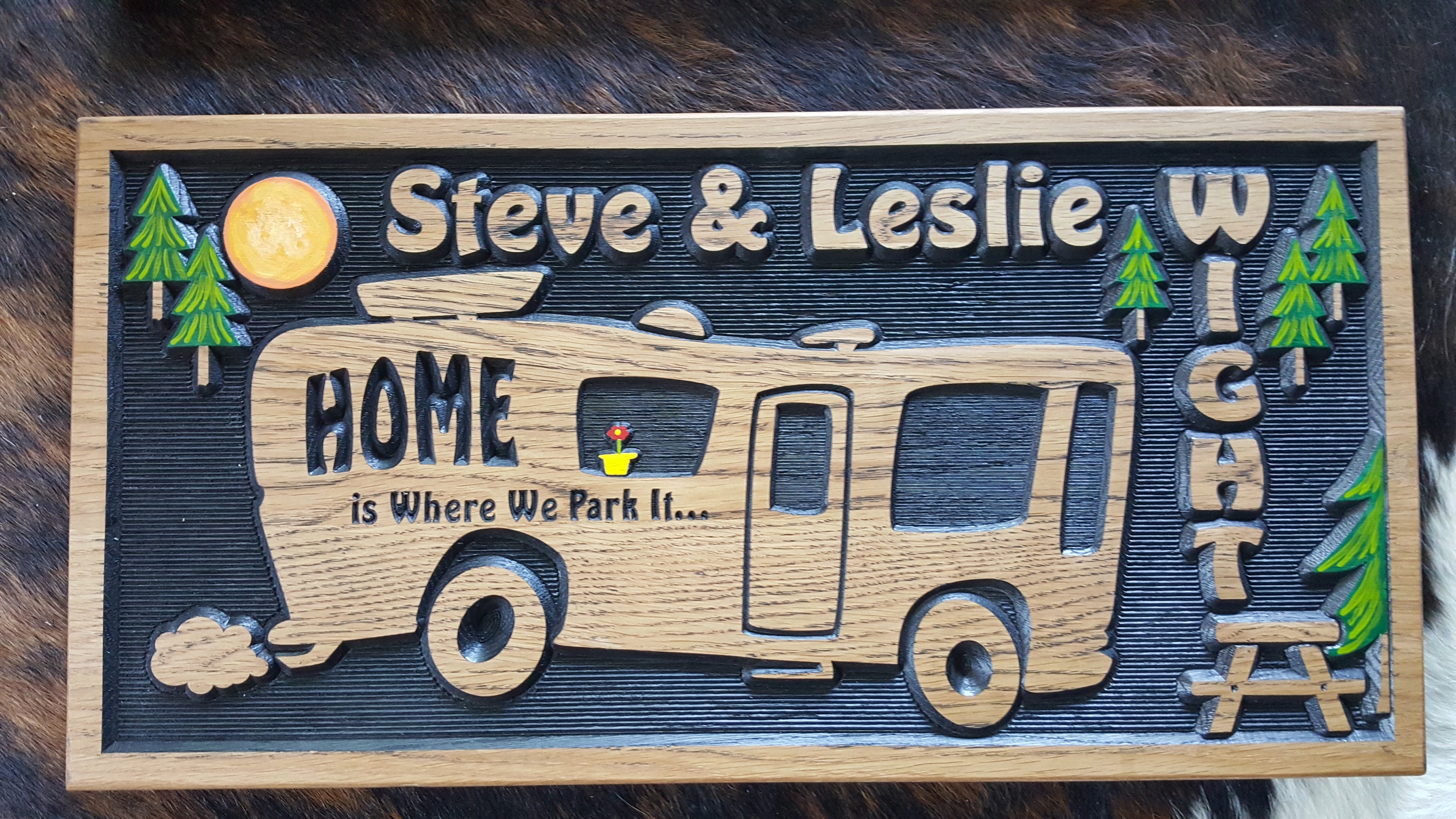The image depicts a meticulously carved wooden plaque dedicated to Stephen Leslie White. Central to the plaque is an RV with intricate details such as a yellow flower pot holding a red flower in its window and whimsical smoke coming out of its exhaust pipe. The plaque features the text "Stephen Leslie White" prominently, followed by the phrase "Home is where we park it." Surrounding the RV are lush green pine trees, shaped like traditional Christmas trees, adding a touch of festive charm to the scene. The bottom right corner of the plaque includes a picnic table, emphasizing a sense of outdoor adventure. The sign also incorporates elements like a sun in the top left corner, creating a warm and inviting feel. The plaque's overall color palette consists of natural wood tones, with accents of black, brown, green, yellow, and red, giving it a rustic appeal. The background appears to be a fir surface, suggesting that the sign might be displayed on a wooden wall or a similar backdrop. Centered and framed, the photograph captures the essence of a lovingly crafted sign that celebrates a lifestyle of freedom and mobility.